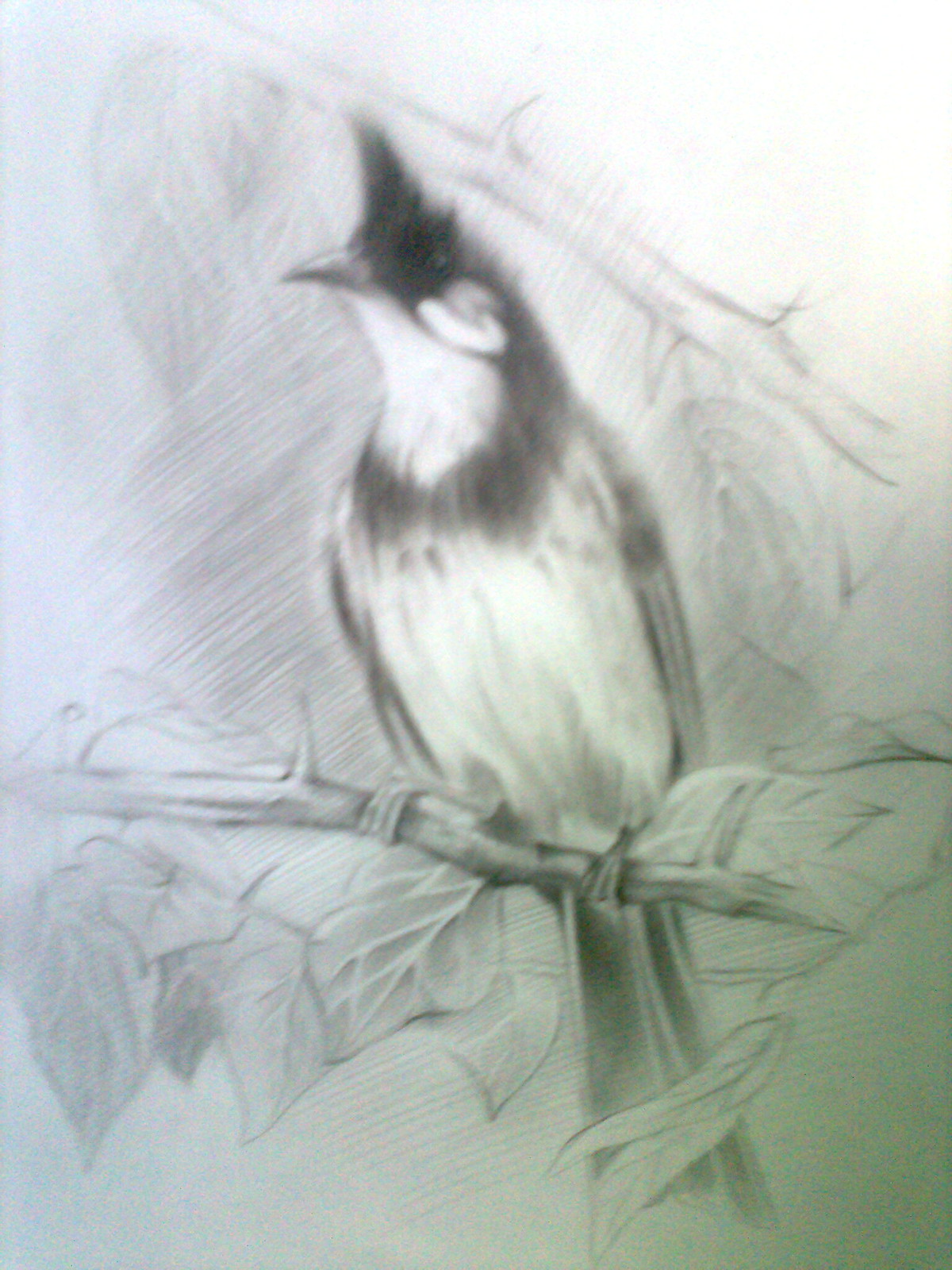This detailed, monochromatic pencil or charcoal drawing depicts a striking bird perched on a thorny branch. The bird features a light-colored underbelly and neck, which contrasts sharply with its darker plumage on other parts of its body. Its sharp, pointed beak and the distinctive crest of feathers resembling a mohawk on its head add to its bold appearance. The intricate textures and careful shading highlight the bird's elegant form against the stark, minimalist background, capturing a moment of natural beauty in exquisite detail.